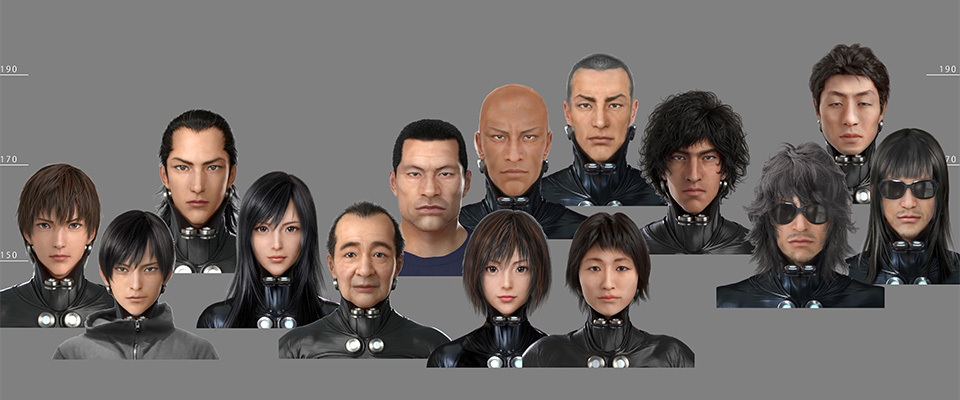The image showcases fourteen animated characters, predominantly male, each depicted from the chest up, with their heads and distinctive hairstyles clearly visible. All characters are presented as if originating from a video game, emphasizing their unreal, digital nature. Among them, there is a diversity: some characters wear black leather jackets, while the man at the center stands out in a blue round-collar t-shirt. Facial accessories like black sunglasses adorn some, particularly the long-haired men positioned on the left, who are around the 150 to 170 height markers on the vertical measurement scale displayed on both sides of the image. These scales, ranging from 150 at the bottom to 190 at the top, further underscore the approximate heights of the characters. The overall setting is enhanced by a gray background, providing a neutral stage for these varied digital personas, which include both men and women, bald and long-haired figures, some exuding a sinister aura while others appear more benign.